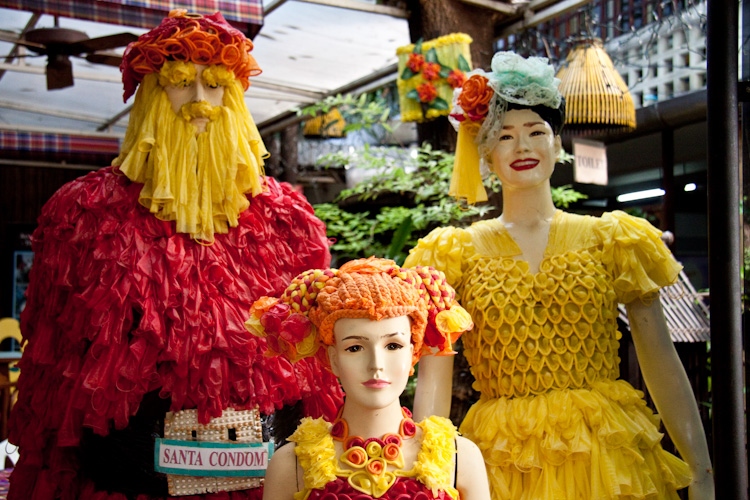In this vibrant full-color square photograph, three mannequins stand prominently, seemingly in a store with shelves and plants visible in the backdrop. The central figure, a young girl, dons spaghetti straps and wears an intricate orange headgear paired with a floral necklace. At her right is an older woman dressed in a long white dress embellished with floral designs and a stylish blue hat. On the left, a man sports an eccentric look with a yellow beard and mustache made from condoms, a pink and orange hat adorned with circular condom ends, and a red shirt with a "Santa Condom" banner across his belly. Each mannequin's outfit incorporates creative floral decor crafted from colorful condoms in hues of yellow, red, and orange, adding a whimsical and intriguing element to the display.